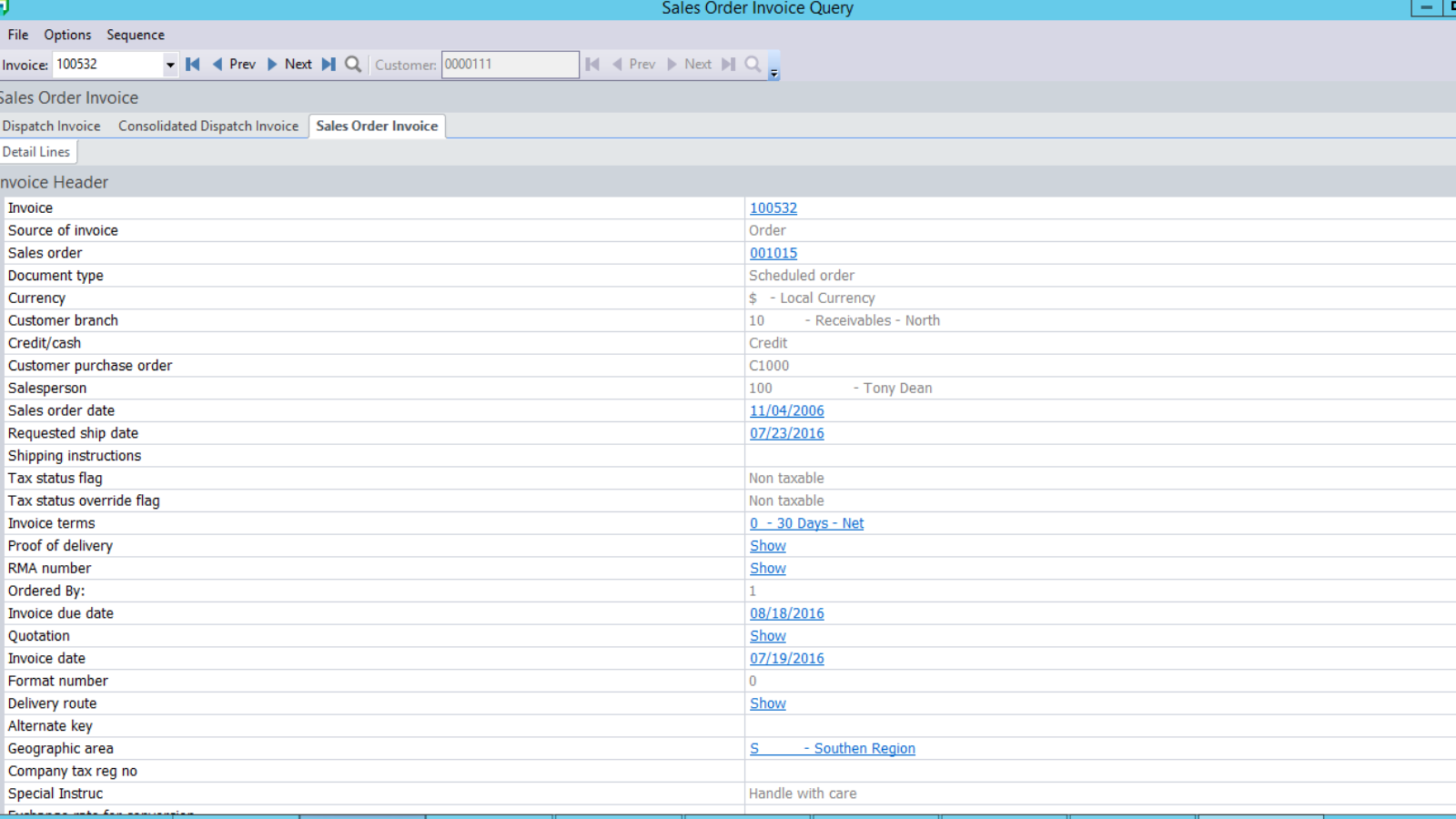The image depicts a software screen titled "Sales Order Invoice Query," prominently displayed on a blue bar at the top. Directly beneath this blue bar are three buttons aligned on the left side labeled as "File," "Options," and "Sequence." 

A gray bar is positioned below this row of buttons, featuring an input field showing "Invoice 100-532" within a white text box. Adjacent to this field are several navigation and search icons, including a back button, another back button, a forward arrow, a fast forward arrow, and a magnifying glass. Below this section, there is another gray bar, although slightly different in color, wih the text "Sales Order Invoice" aligned to the left. 

Furthermore, this gray bar hosts three tabs: "Dispatch Invoice," "Consolidated Dispatch Invoice," and "Sales Order Invoice," enabling the user to navigate between different invoice views or functions. The detailed arrangement and labeling make it a concise and well-structured interface for managing and querying sales order invoices.